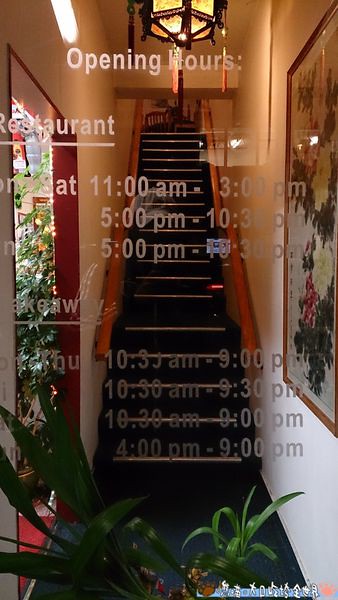The photograph is a color image in portrait orientation, capturing an interior view into a restaurant through a piece of glass that displays the restaurant's opening hours in white text. The scene focuses on a staircase with a dark wood finish and medium-toned handrails on either side, leading upward. Black carpeting lines the stairs, and at the base, a green plant with visible leaves stands out. Overhead, a wrought iron light fixture with tassels hangs, casting light into the foyer-like entrance. The white walls are adorned with framed floral artwork on the right, while to the left, there is a doorway with red carpeting leading into another space. Additional fluorescent lighting is visible on the left, enhancing the overall illumination. The opening hours are detailed in white font on the glass: "11 a.m. to 3 p.m. and 5 p.m. to 10:30 p.m." with other hours stating "10:30 a.m. to 9 p.m. and 4 p.m. to 9 p.m." A light blue strip with white script and foreign lettering appears at the bottom right corner, adding to the photographic realism and representationalism style of the image.